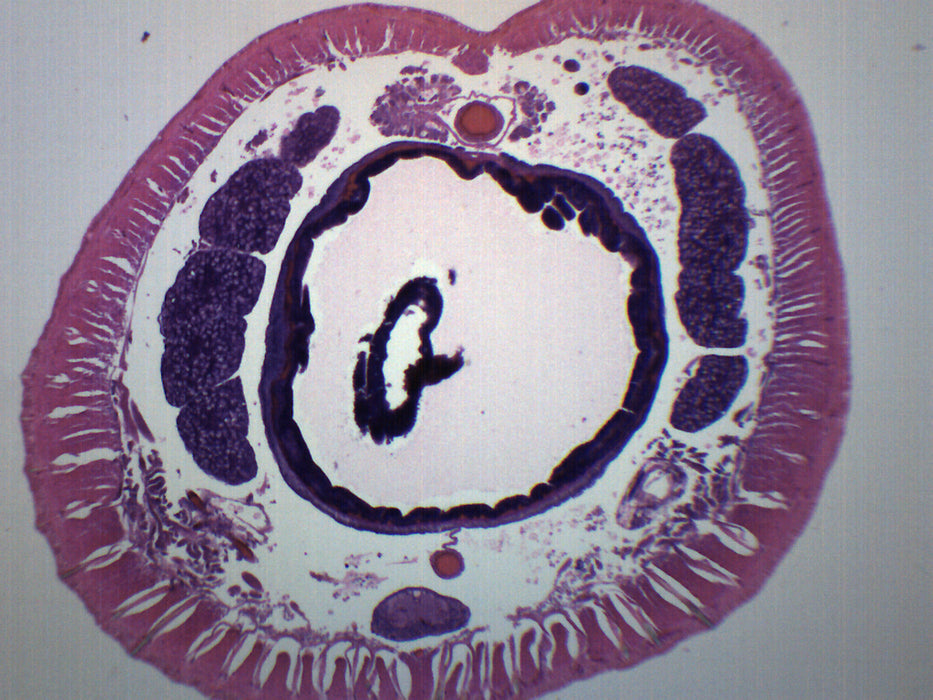The image depicts a detailed microscopic scan of a tissue sample, possibly of brain tissue. The tissue is showcased in a side cutaway view, revealing a complex structure. The exterior is pink, forming an outline that is heart-shaped or resembles a tomato. Just inside this outer layer, there is a mid-layer dotted with purple blobs and blotches. The most striking feature is a central dark purple ring that surrounds an oblong, vertically oriented nucleus-like structure with a white center. This central nucleus is speckled with black spots and purple dots. Additionally, at the bottom of the image, there appears to be a structure resembling a sperm cell, with a prominent round head and a tail. The background of the image is a light gray, which contrasts with the vivid colors of the tissue, emphasizing the intricate organic patterns and cellular details within.